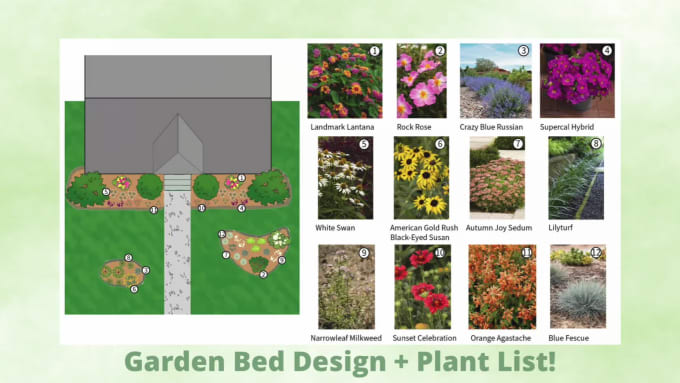This photograph captures a detailed flyer titled "Garden Bed Design and Plant List." On the left side, there's a bird's eye view diagram of a garden layout adjacent to a house and driveway, complete with trees in the yard. The right side of the flyer exhibits twelve different samples of various kinds of foliage, mostly flowers, displaying gardening options within your grass. Although the text naming the plant types, such as 'Landmark Lantina' and 'Crazy Blue Russian,' is blurry and hard to read, the diversity of plants is clear. The flyer itself is in shades of green, appearing delicate and possibly sourced from a rest area laden with similar advertisements.